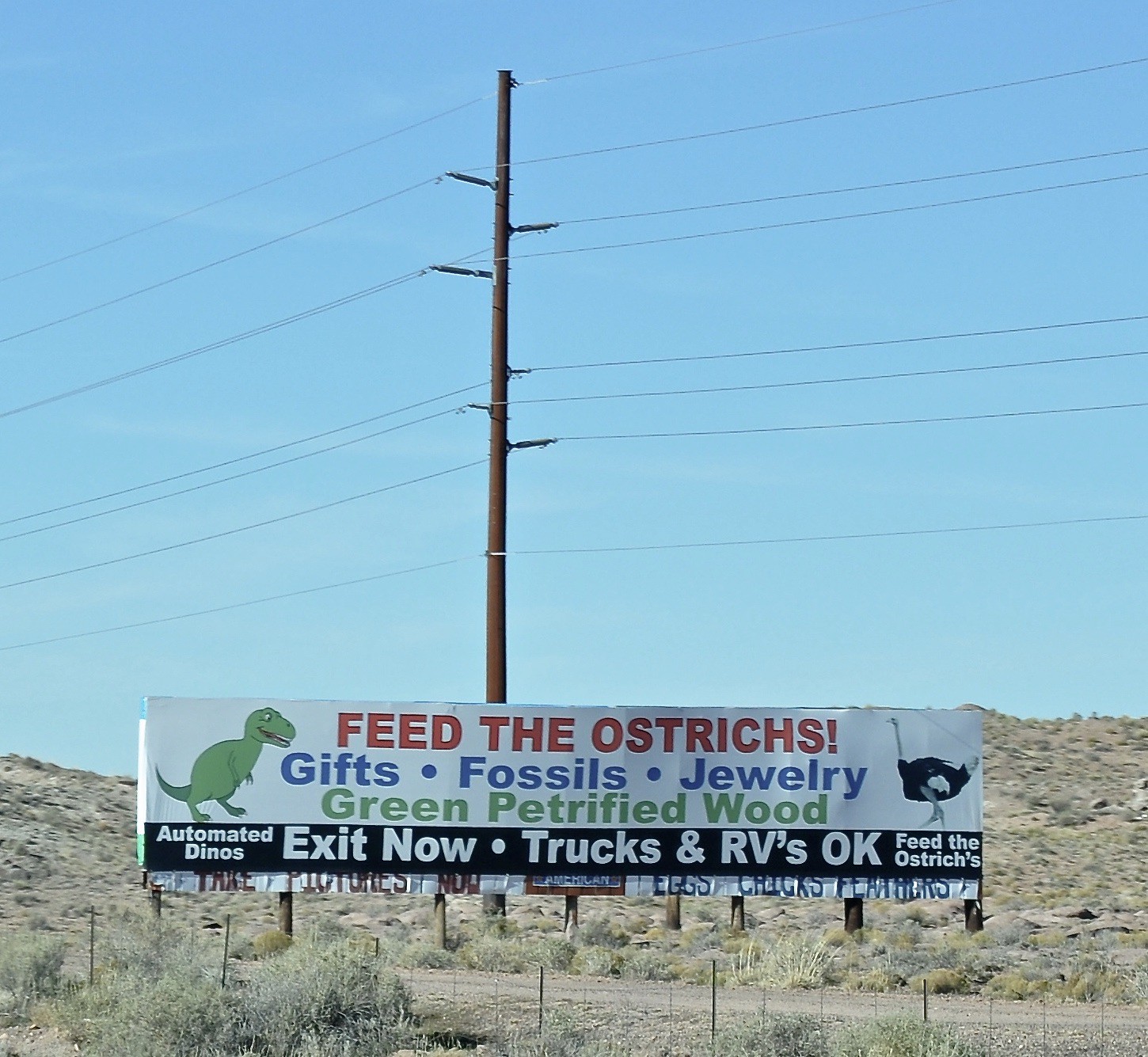The photograph captures a square image focusing on a roadside billboard, seemingly in a dry, desert-like area possibly in the southern United States near Mexico. The background features a bluish sky with thin, distant clouds, and rolling hills dotted with sagebrush and small vegetation patches.

The prominent billboard, situated by a dirt road, is largely white with a black border at the bottom. On the white section, bold red lettering advertises, "feed the ostriches," despite a misspelling, along with listings for gifts, fossils, jewelry, and green petrified wood. The left side of the billboard highlights an illustrated green dinosaur, resembling a Tyrannosaurus rex, while the right side showcases an ostrich. 

Below, on the black border, the text "automated dinos, exit now, trucks and RVs okay, feed the ostriches" is clearly displayed. There's additional text about taking pictures and acquiring eggs, chicks, and feathers, presumably ostrich-related.

A large wooden telephone pole stands tall in front of the billboard, radiating a complex web of many wires, secured with multiple connectors. A fragment of fence and rough terrain with brown soil and sparse greenery extend towards the horizon, emphasizing the remote, arid setting of this roadside attraction.